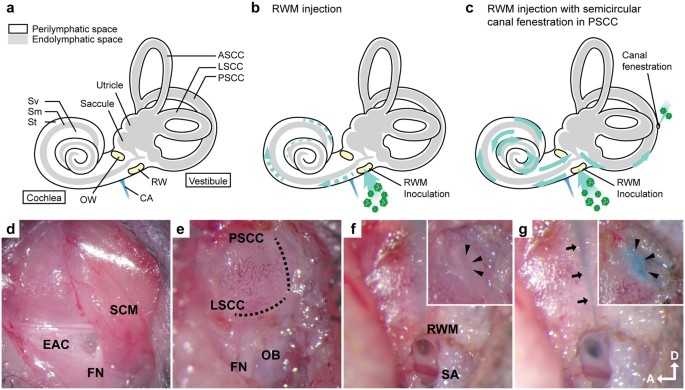This comprehensive medical illustration presents detailed anatomical and procedural images of the human ear, specifically focusing on the cochlea and the semicircular canals. The top row features three schematic diagrams labeled 'A,' 'B,' and 'C,' illustrating various anatomical structures such as the perilymphatic and endolymphatic spaces, utricle, saccule, and different parts of the semicircular canals (ASCC, LSCC, PSCC). These diagrams also highlight distinct procedures, with labels like 'RWM injection' and 'RWM injection with semicircular canal fenestration in PSCC.'

The bottom row consists of four real-life microscopic photographs labeled 'D,' 'E,' 'F,' and 'G' that show the interior of the ear, marked by their vivid, pinkish flesh tones indicating live tissue. These images provide a graphic, close-up view of the ear’s internal organs, mirroring details from the diagrams above. The juxtaposition of the clinical schematics with the visceral tissue images offers a comprehensive visual study of ear anatomy and medical interventions, enhancing understanding of complex ear structures and surgical procedures.